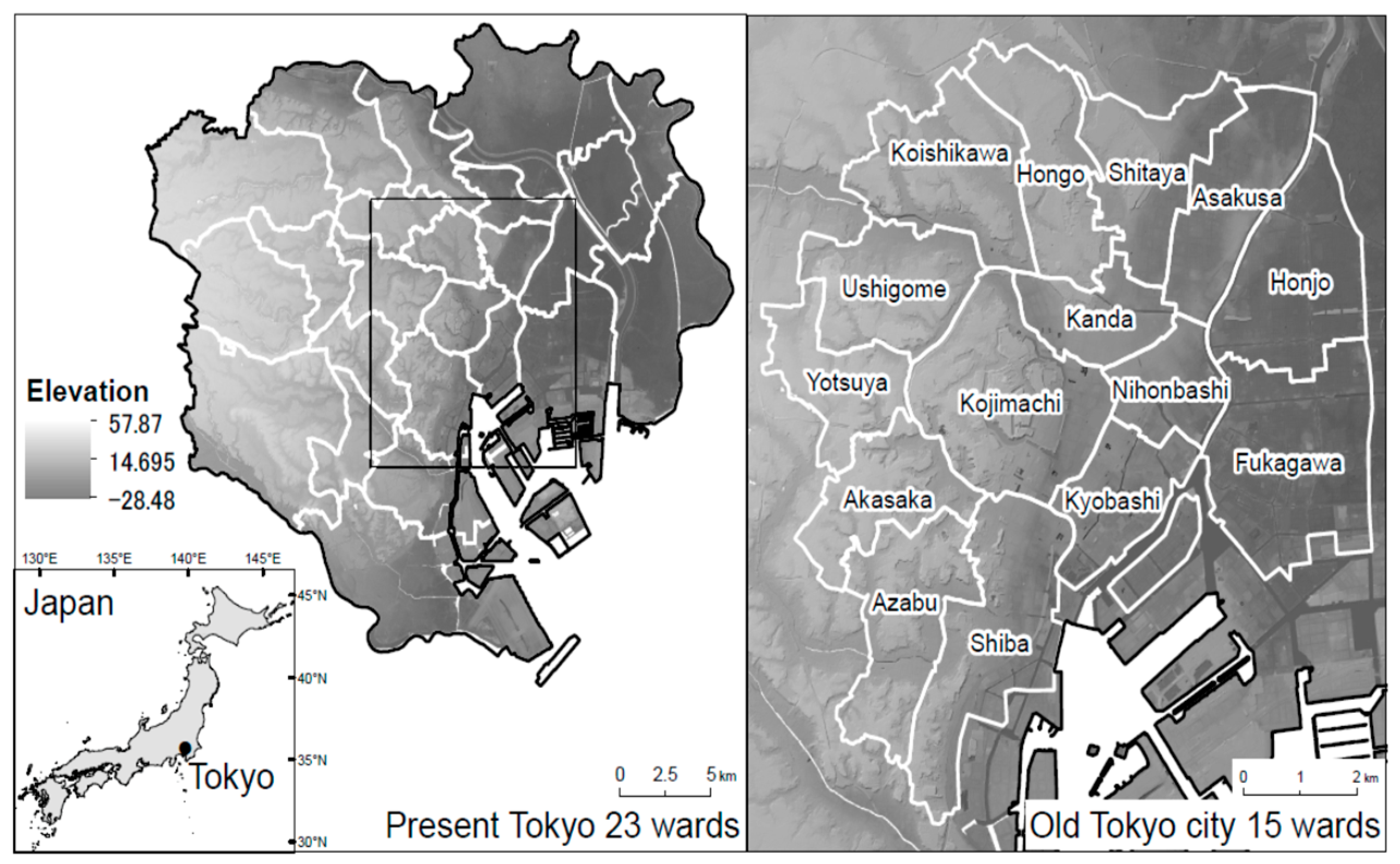This image presents a detailed comparison between present-day Tokyo and old Tokyo City through two juxtaposed maps. 

The left half displays a grayscale map labeled "Present Tokyo, 23 Wards," featuring the current metropolitan layout of Tokyo. This map includes an inset showing the entire outline of Japan, faintly shaded in light grey, with Tokyo pinpointed. It vividly represents different elevations, transitioning from dark grey for lower areas to light grey for higher elevations, indicated by a vertical bar graph with markers at -28.48, 14.695, and 57.87. Additionally, Tokyo Bay is partially showcased within a square overlay highlighting a particular section of the city. A scale for distances denoted in kilometers (0, 2.5, and 5 km) is also present, enhancing the map's practical detail.

On the right side, the map titled "Old Tokyo City, 15 Wards" focuses on historical Tokyo, outlining the 15 wards with geographic borders and names in black font against a white outline. This map similarly uses a grayscale gradient to represent elevation differences and includes a distance scale marked from 0 to 2 kilometers. The names of the historic wards—Koishikawa, Hango, Shitaya, Asakusa, Hango, Kanda, Ushigomi, Yotsuya, Kojimacha, Nihonbashi, Fakagawa, Kayobashi, Shiba, Azuba, and Akasaka—are clearly mapped, emphasizing the municipal divisions of the past.

Overall, the image provides a comparative analysis of Tokyo's urban evolution, contrasting present-day Tokyo's 23 wards with the 15-ward structure of old Tokyo City, highlighted through detailed grading, geographic markers, and elevation representations.